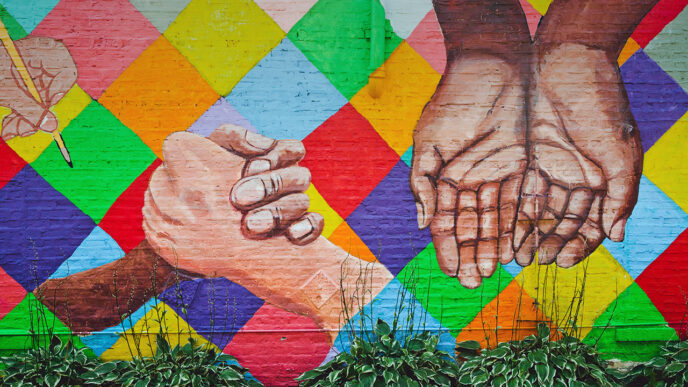The mural, painted vividly on a brick wall, encapsulates themes of community, equality, and friendship. It features a diagonal crisscross pattern with an array of colors, including shades of green, yellow, red, blue, orange, pink, light blue, and gray, creating a quilt-like background. On the left side, a hand holding a pencil suggests the act of creation or storytelling. Adjacent to it, two hands—one brown and one white—grasp each other in a firm handshake symbolizing unity and solidarity. Further to the right, two brown hands are cupped together, palms facing outward as if in an offering gesture. The mural’s intricate design is further enriched by the background's checkered pattern, hinting at a message of peace. Below the mural, a few plants add a touch of natural beauty to the scene.